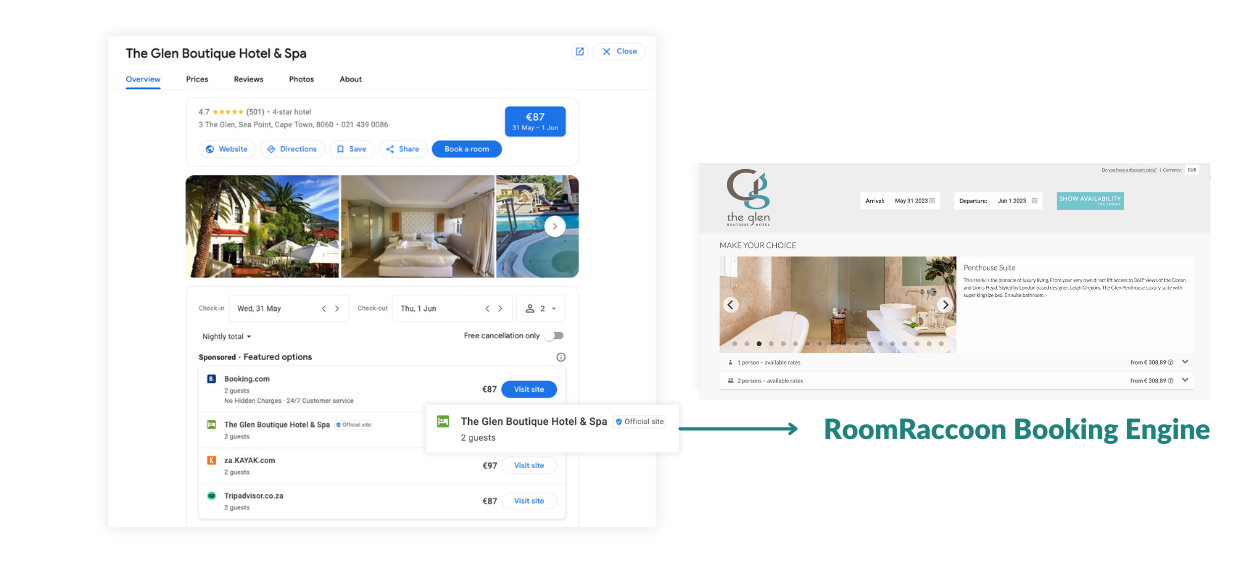The image displays two side-by-side screenshots, each providing a glimpse into different digital representations of the Glenn Boutique Hotel and Spa. 

On the left side, the screenshot features a website with a white background, indicating an online travel booking platform, potentially Expedia or Booking.com. In the top left corner, "The Glenn Boutique Hotel and Spa" is prominently displayed. Below this, a navigation menu in blue lists options: Overview, Prices, Reviews, Photos, and About. The establishment boasts a remarkable 4.7-star rating, as discerned from the gold stars next to an extensive number of reviews, although the exact count is too small to be legible. Beneath the rating, three photos provide a visual tour of the hotel. The first image on the left showcases the hotel's exterior with a white façade, surrounded by palm trees and set against a clear blue sky. The central image captures the interior of a hotel room, featuring a large bed with a white comforter and a notable large window to the left. The third image on the right illustrates a poolside scene.

The screenshot on the right presents what appears to be the hotel’s official website, also set against a white background. This site’s header is gray, displaying a sleek logo comprised of a stylized gray "G" and "B." Beneath the logo, the name "The Glenn" is emphasized, followed by the tagline "meet your choice." The main photo within this screenshot likely depicts a serene spa environment, highlighting a luxurious jacuzzi tub on one side and an adjacent countertop, suggesting a space designed for relaxation and tranquility.